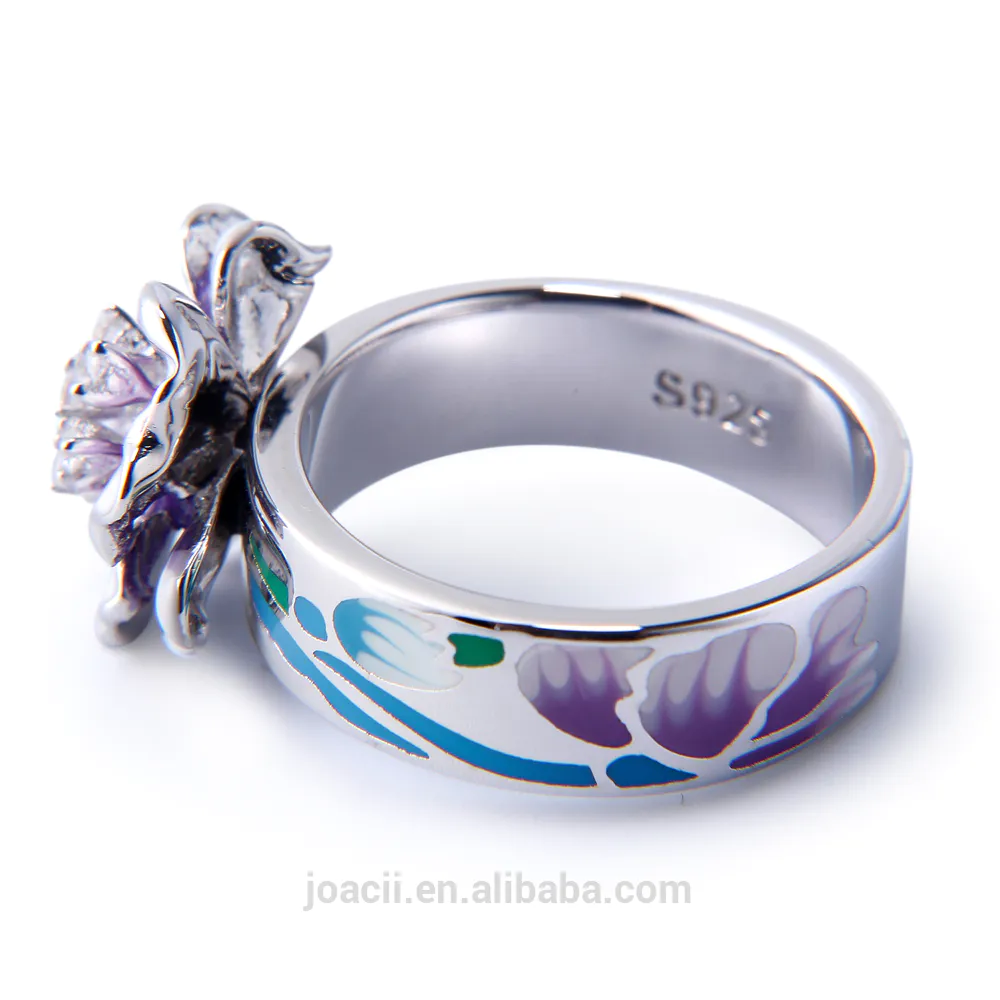This image, sourced from joaci.ien.alibaba.com, features a close-up view of a lady's silver ring, engraved with "S925" on the inside, indicating its silver composition. The ring is shown lying on its side, allowing a detailed view of its elaborate design. The ring's exterior appears to have a white ceramic-like coating, adorned with various shapes in blue, purple, and green hues that accentuate its appearance. On the top left of the ring is a prominent silver flower design, with hints of purple detailing. This flower may also encase a diamond or gemstone, although it's partially obscured and difficult to discern clearly. The ring is relatively small and the image is zoomed in to highlight intricate details, suggesting a custom-made piece with a thick band that stands out due to its colorful and artistic design elements.